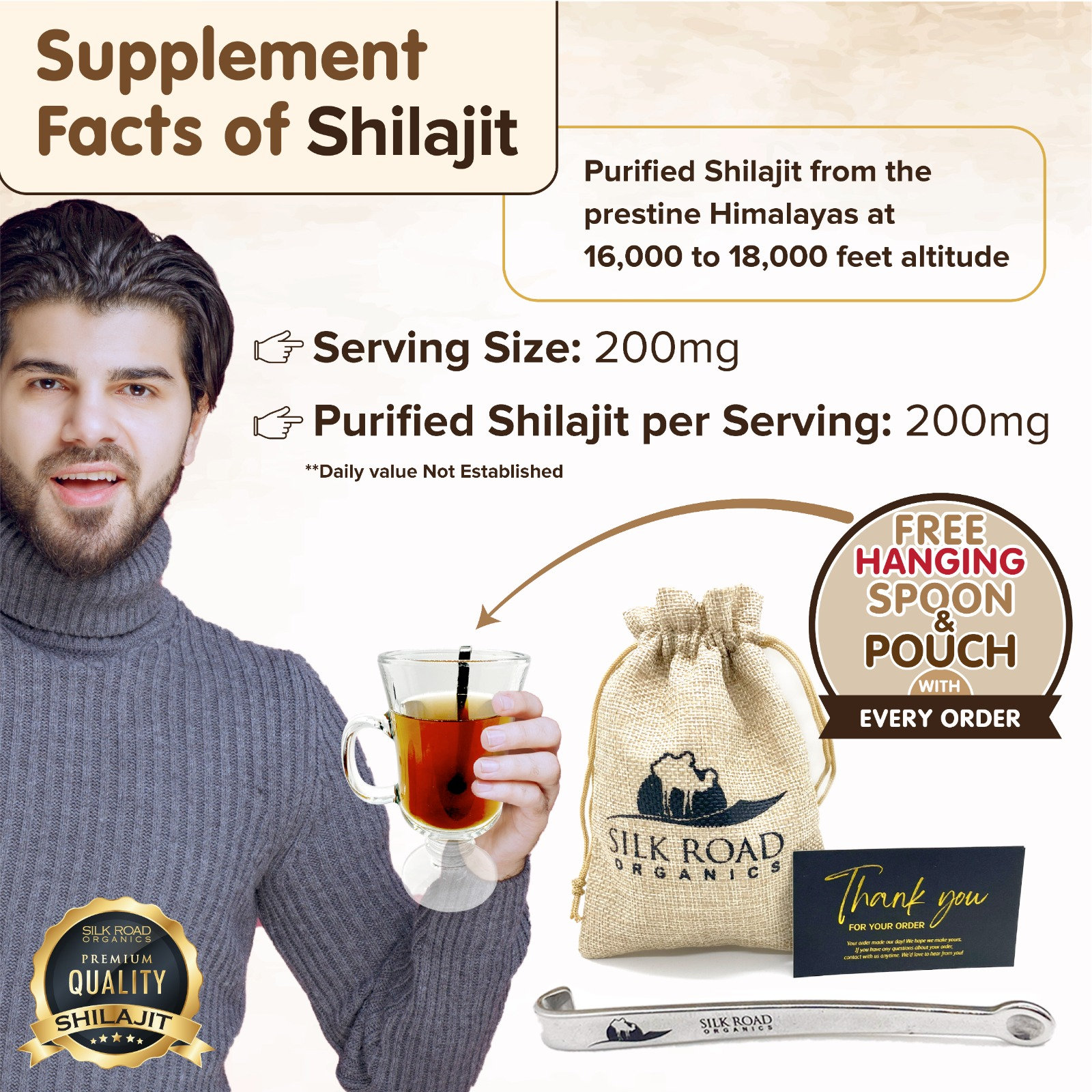The image is a detailed advertisement for Silk Road Organics' Shilajit supplement. The ad prominently features a gentleman in a blue turtleneck sweater holding a clear glass of tea-like Shilajit, complete with a small black straw. The text details the supplement facts, stating that it contains purified Shilajit sourced from the pristine Himalayas at altitudes ranging from 16,000 to 18,000 feet, with a serving size of 200 milligrams. The ad highlights that each order includes a free hanging spoon and a pouch emblazoned with the Silk Road Organics logo, which features a camel and a stylized background. Adding to the premium feel, there is a seal of approval indicating premium quality, and a black and gold card saying "Thank you for your order." The complimentary spoon, also branded with Silk Road Organics, is prominently displayed near the burlap pouch.